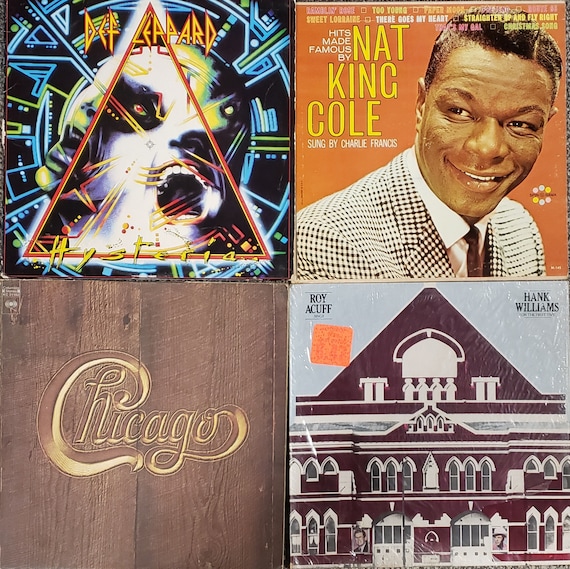This image showcases the covers of four distinct vinyl albums, each square-shaped, representing iconic artists. 

In the upper left, the Def Leppard "Hysteria" album features a bold red triangle framed by dynamic blue and green lines, set against a black background with futuristic elements. To the right, the upper right cover displays Nat King Cole's classic album "Hits Made Famous by Nat King Cole" sung by Charlie Francis. The cover is an orange backdrop with a yellow font, showcasing a smiling Nat King Cole dressed in a sophisticated black and white checkered overcoat, white shirt, and tie.

The bottom left features Chicago's famous self-titled album, "Chicago," characterized by a dark brown wooden plank design that highlights its intricate wood grain, with the band name artistically scripted in gold.

Lastly, the lower right album cover belongs to Roy Acuff and Hank Williams. It presents a maroon-red architectural structure with white accents and a pointed roof. The names "Roy Acuff" and "Hank Williams" appear in the upper corners, with small photographs of the artists in the building's windows.

Together, these album covers exemplify a range of musical genres and artistic styles, from rock and jazz to country, each capturing the essence of their respective artists.